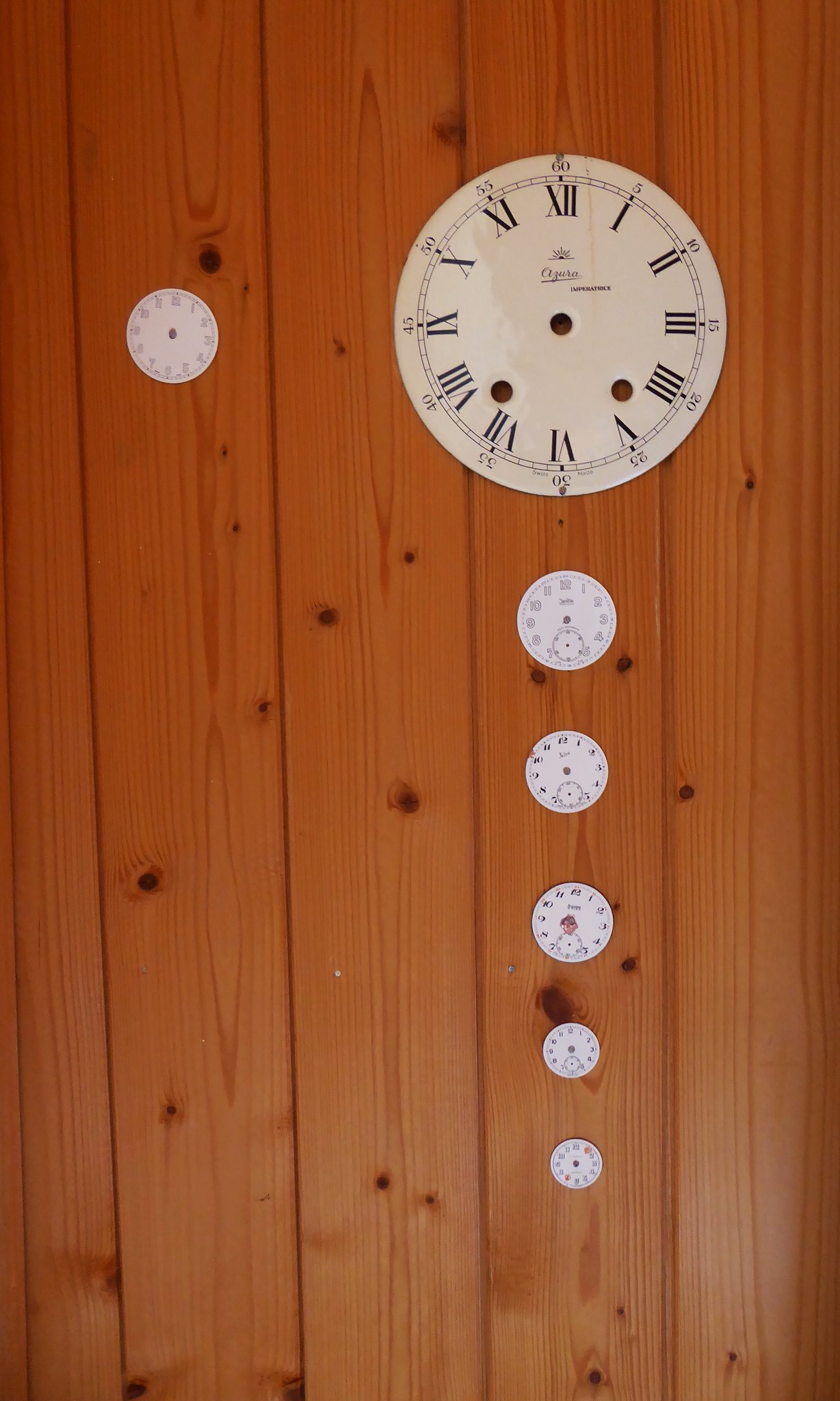The image portrays a light brown wood-paneled wall adorned with seven paper clocks, each meticulously arranged. The most prominent feature is a large paper clock situated on the second plank from the right, distinguished by its Roman numerals and lack of clock hands. Below this dominant clock, five smaller clocks are sequentially arranged, decreasing in size as they descend the plank. On the second plank from the left, there's an additional small paper clock. The wood paneling, marked by subtle dark specks, consists of five visible vertical planks, providing a rustic backdrop to the clustered display of the handless clocks. The overall composition appears as if the clocks are simply faces adhered to the wall, exuding an impression of static time.